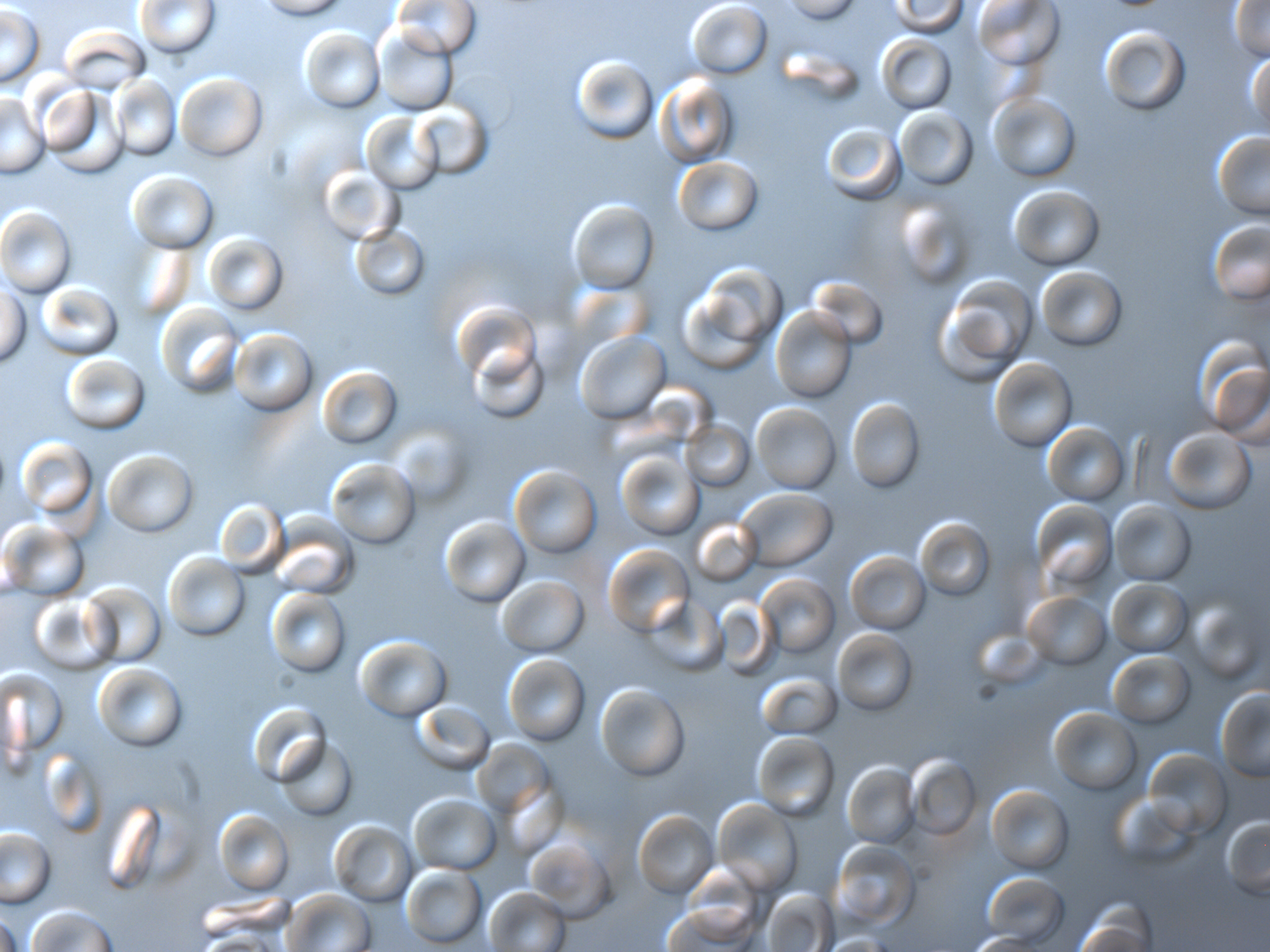This image, appearing to be taken under a microscope at an extreme close-up level, depicts a dense field of semi-transparent, gel-like circular orbs resembling white blood cells. The slightly bluish-gray background is filled with numerous bubble-like structures, each possessing a circular or doughnut shape with a divot in the center. Among the sea of orbs, which number well over 100, some exhibit a faint apricot-peach tint and a prominent specular highlight, adding to their three-dimensional appearance. The background is softly blurred, creating a contrast with the more sharply focused orbs, though some are slightly rotated and out of focus, particularly near the edges. The overall color palette is a mixture of light blue, gray, and off-white hues, emphasizing the delicate and intricate nature of the microscopic scene.